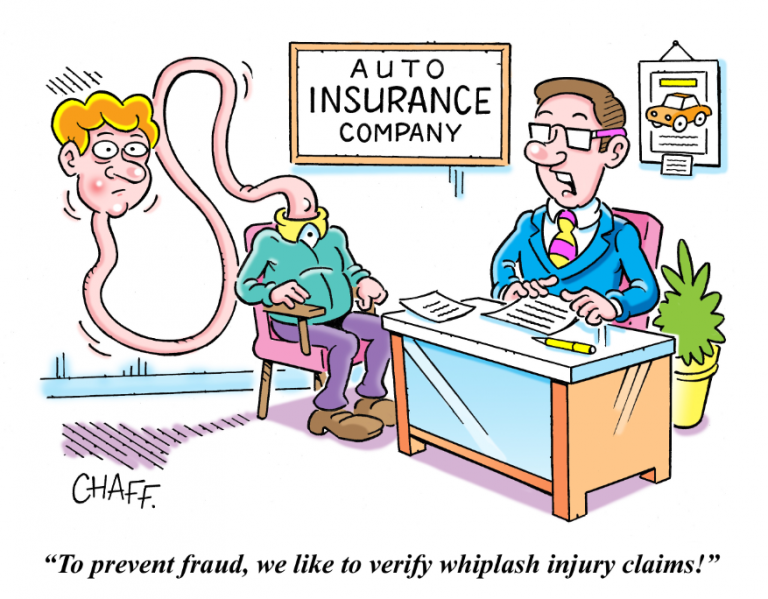The image is a humorous and satirical cartoon set inside an auto insurance company office. The setting is clearly indicated by a sign on the wall that reads, "Auto Insurance Company." Behind a desk, a man in professional business attire is conversing with a client whose neck is exaggeratedly long, practically looped and dangling like a snake, emphasizing a severe whiplash injury. The client sits in a pink chair with a pained expression, his head nearly across the room, creating a comical yet poignant scene. A framed photo also hangs on the white wall, adding to the office atmosphere. The quote at the bottom of the image humorously states, "To prevent fraud, we like to verify whiplash injury claims," pointing to the absurd length the insurance company goes to verify claims. The artist's signature, "CHAF," is neatly placed at the bottom left corner.